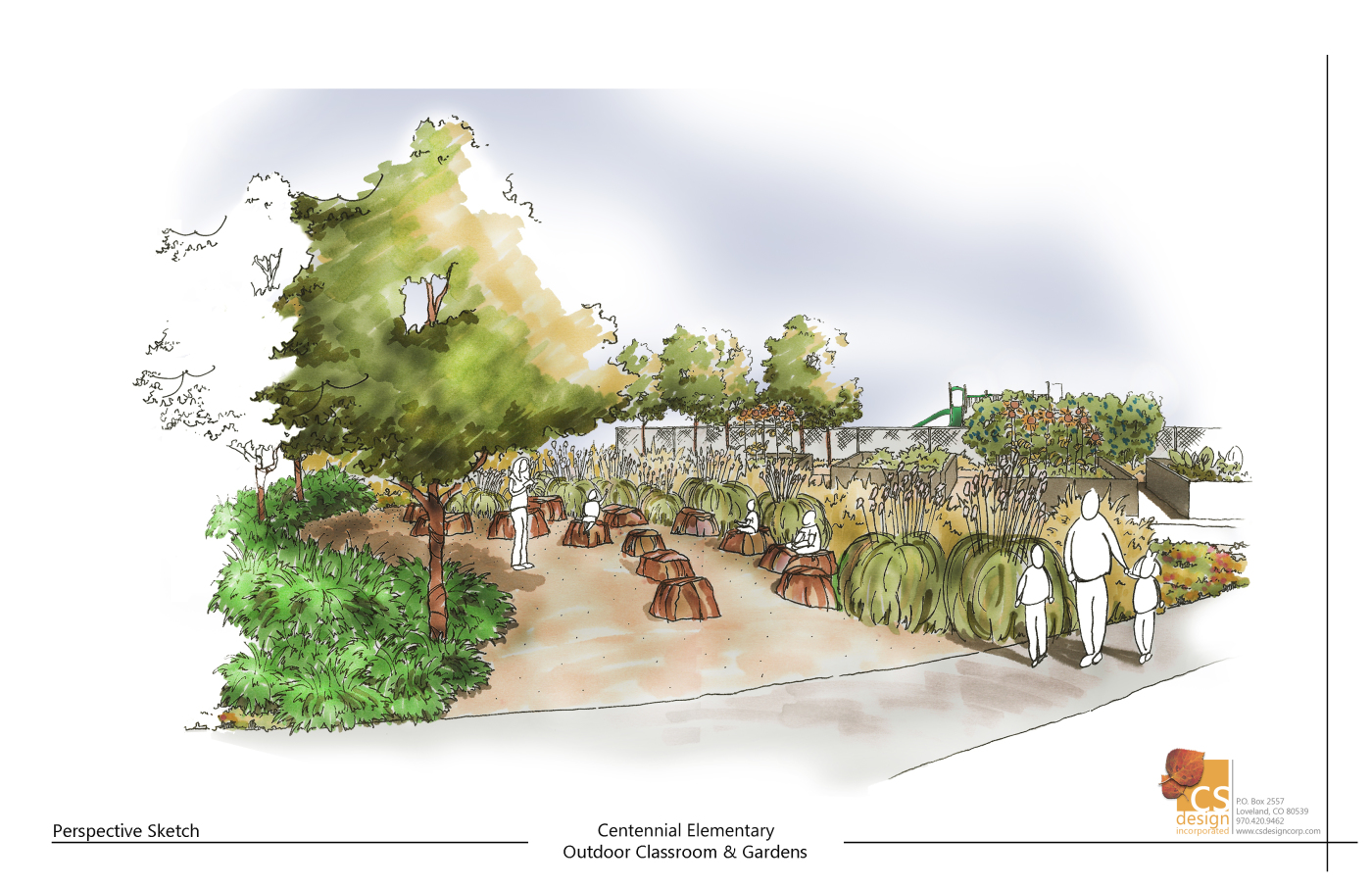The image portrays a detailed, colored sketch of "Centennial Elementary Outdoor Classroom and Gardens," as indicated by the text in the middle of the artwork. The bottom left corner of the image reads "Perspective Sketch," while the bottom right corner features an orange leaf artwork followed by the text "CS design," with additional, smaller, unreadable text. Set against a white background, the scene is a vibrant outdoor garden with elements of green grass, trees, and a sidewalk running from left to right. The sketch includes pencil-drawn, faceless figures with white circular heads, outlined in black. Several figures are walking along a path on the right side, while others are sitting on tree stumps and rocks in the center, resembling students in an outdoor classroom. The background features plant life and a distant building, and the overall ambiance is bright and clear, with a few figures engaged in drawing activities. The sketch captures the lively essence of an outdoor learning environment amidst natural greenery and clear lighting.